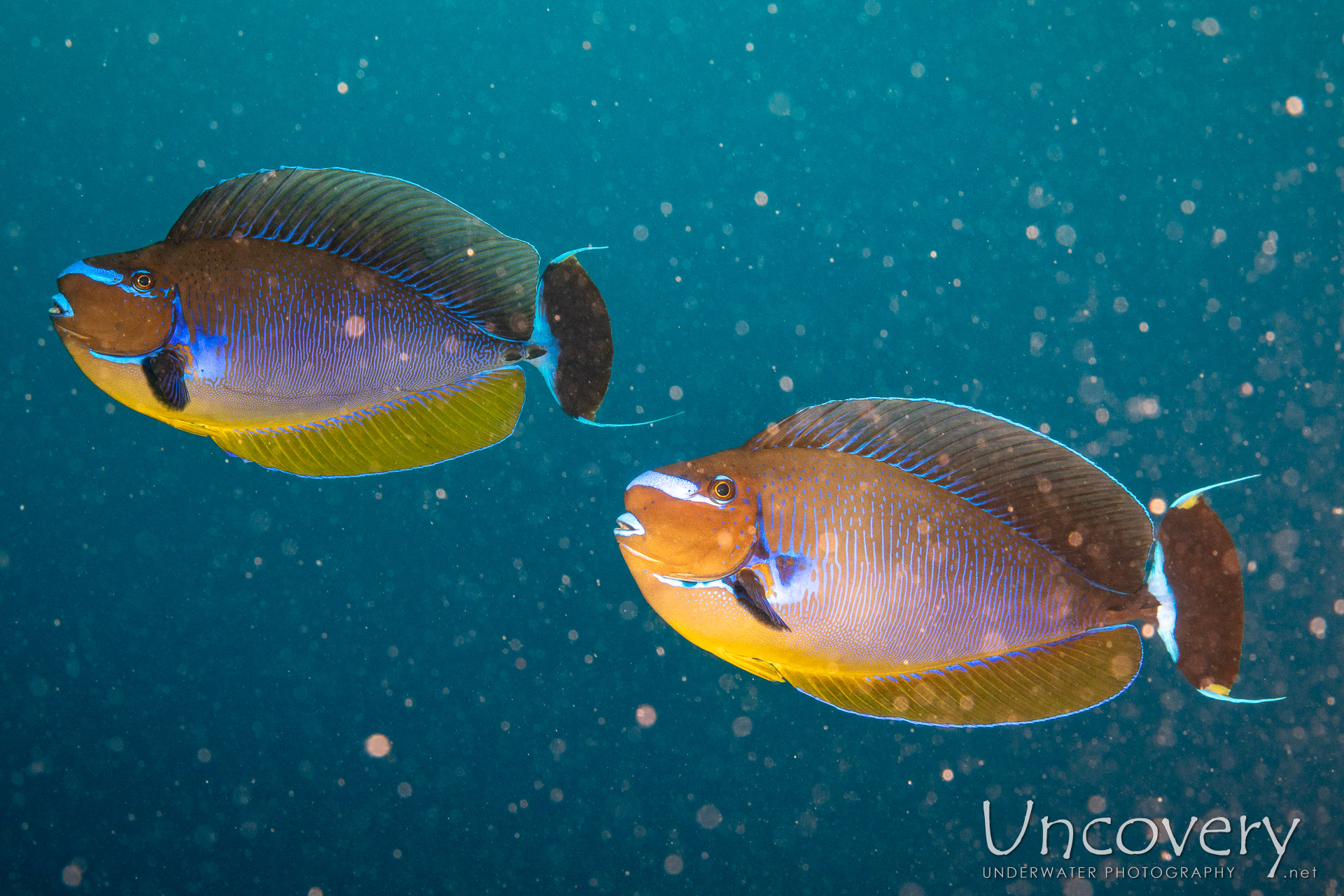This is an artistically rendered underwater scene, showcasing two tropical angelfish swimming in a vibrant, aqua-green ocean. Both fish exhibit a luminous array of colors and are facing towards the left edge of the landscape-oriented frame. The fish on the top left is slightly smaller, adorned with bright blue highlights around its nose and mouth, extending along the base of its fins and scales. Its primary body color is purple, complemented by a dark green dorsal fin and a yellow fin on its underbelly. The tail is black with bright blue, pointed structures.

The larger fish on the right displays a similar body shape but a distinct color palette. It features a white stripe on its forehead and around its mouth, brown on the center of its tail, and white elongated sections at both the top and bottom of its tail. The captivating scene is composed against a serene, deep aqua-blue background, with occasional bubbles hinting at movement and depth.

In the bottom right corner, the text "UNCOVERY" appears prominently, followed by "underwater photography" in smaller white letters. The overall style fuses photographic realism with artistic representationalism, emphasizing the vivid colors and delicate details of the underwater world.